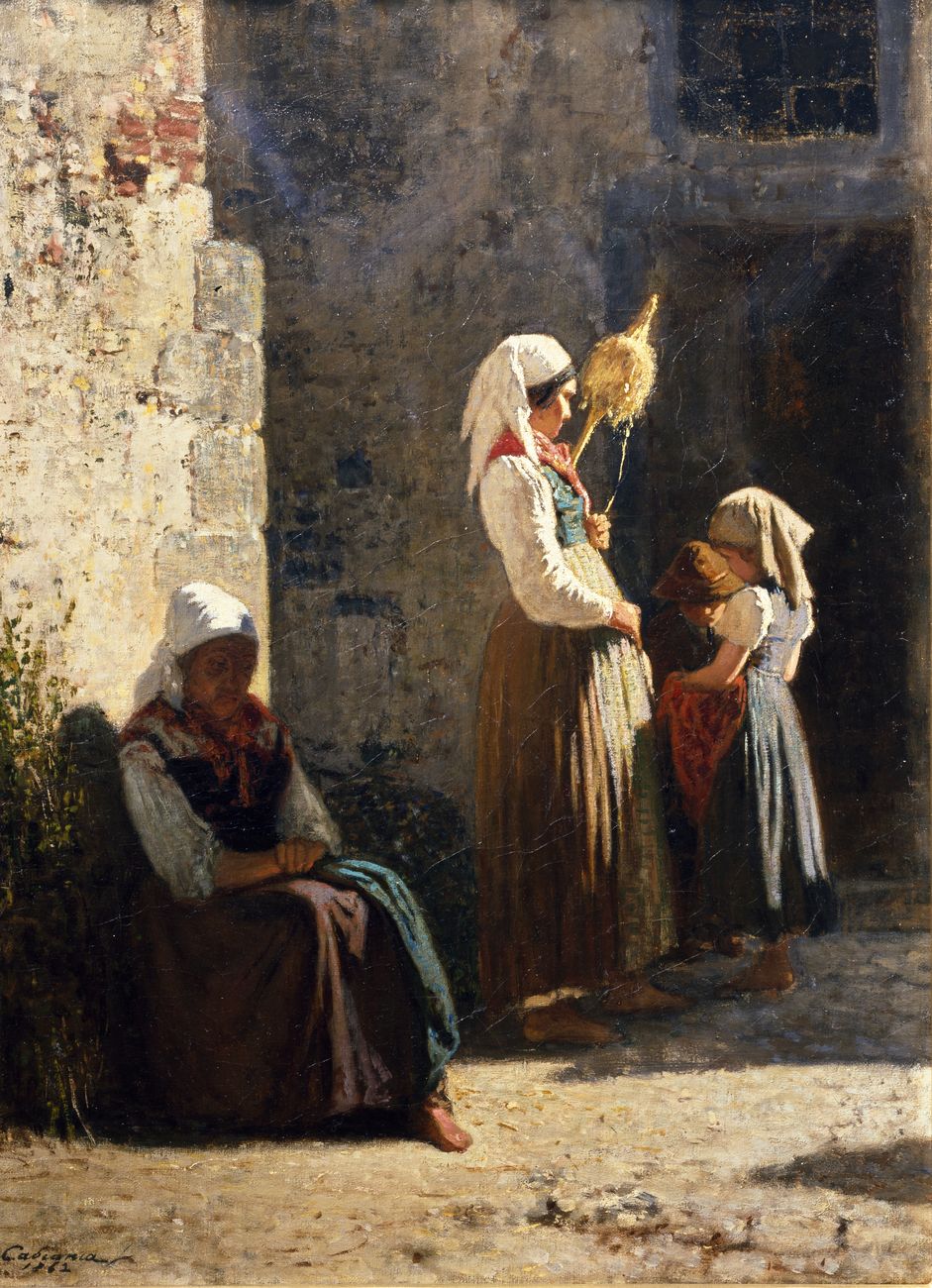The painting depicts a tranquil rural scene with four individuals set against a backdrop of gray and white stone buildings. The cobblestone road underfoot enhances the rustic charm of the setting. On the far left, a woman in a dark red dress over a white blouse sits somberly against a stone wall, her hair tied with a white cloth and a red scarf around her neck. To her right stands another woman, her hand resting on her stomach, dressed in a green dress accented by a green vest and a white shirt, her head covered with a white scarf. Beside this standing woman are two children. One child, positioned slightly behind the other, wears a blue dress with short white sleeves and holds a red cloth. The overall composition is captured in soft sunlight, casting gentle shadows and adding depth to the scene. A small bush grows near the seated woman, and a window is visible on the rightmost building, adding detail to the idyllic rural backdrop.